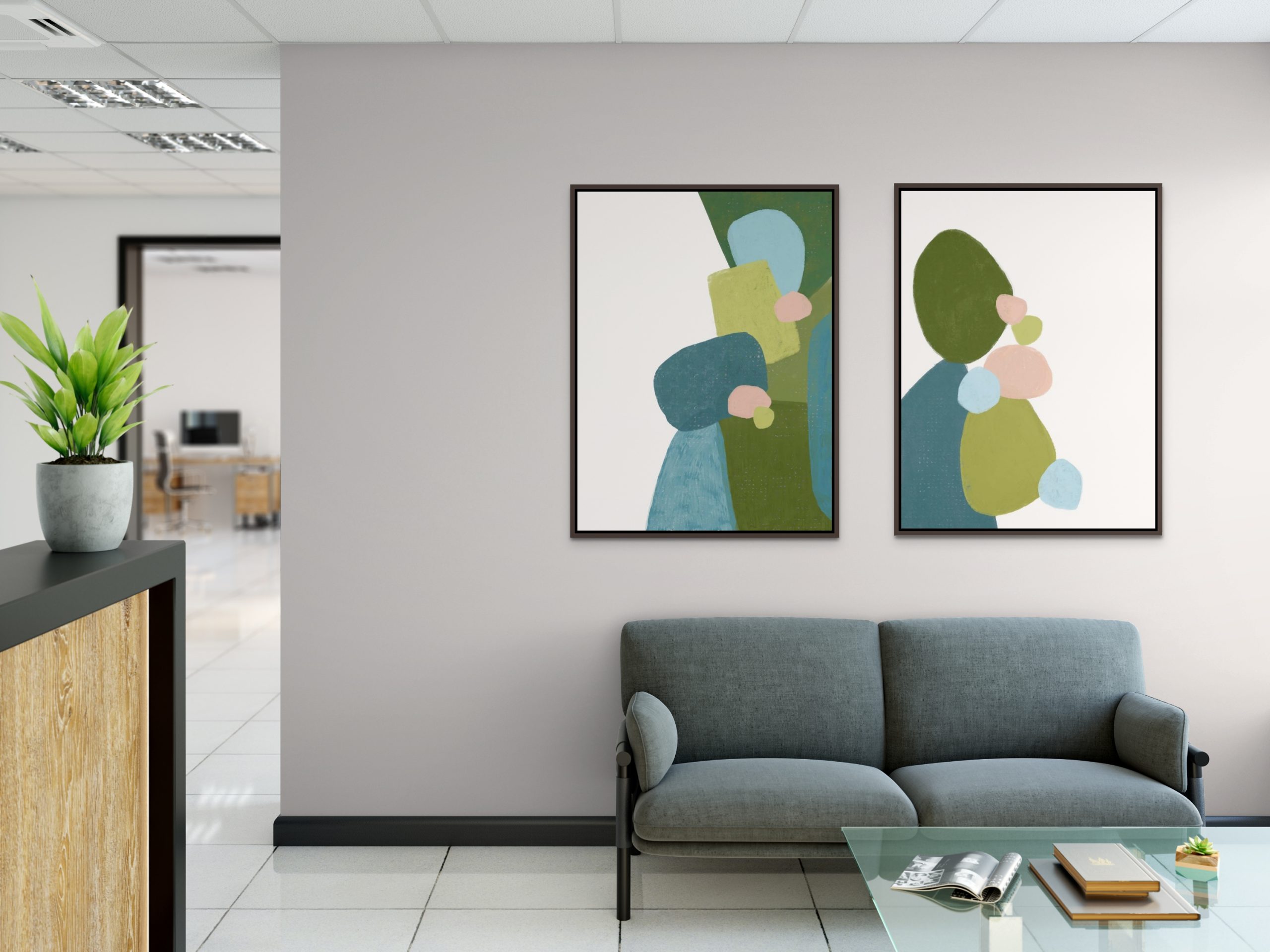The photograph depicts a waiting room, likely in a doctor's office, featuring a neatly arranged seating area. Dominating the right side is a dark gray loveseat with black legs, positioned against a light gray wall accented with black floor molding. Above the loveseat, two abstract paintings with thin black frames hang side by side, displaying various shapes in shades of green, teal, pink, and beige on a white background.

A transparent glass table stands in front of the loveseat, holding an assortment of books and an open magazine. The floor is covered in white tiles. To the left of the image, there is a brown wood-paneled reception desk with a black countertop, adorned with a small, vibrant green potted plant.

In the background on the left, an entryway leads to another room, revealing a computer within. Overall, the image captures a clean, welcoming space designed for patient comfort, with its neutral color palette and modern furnishings.